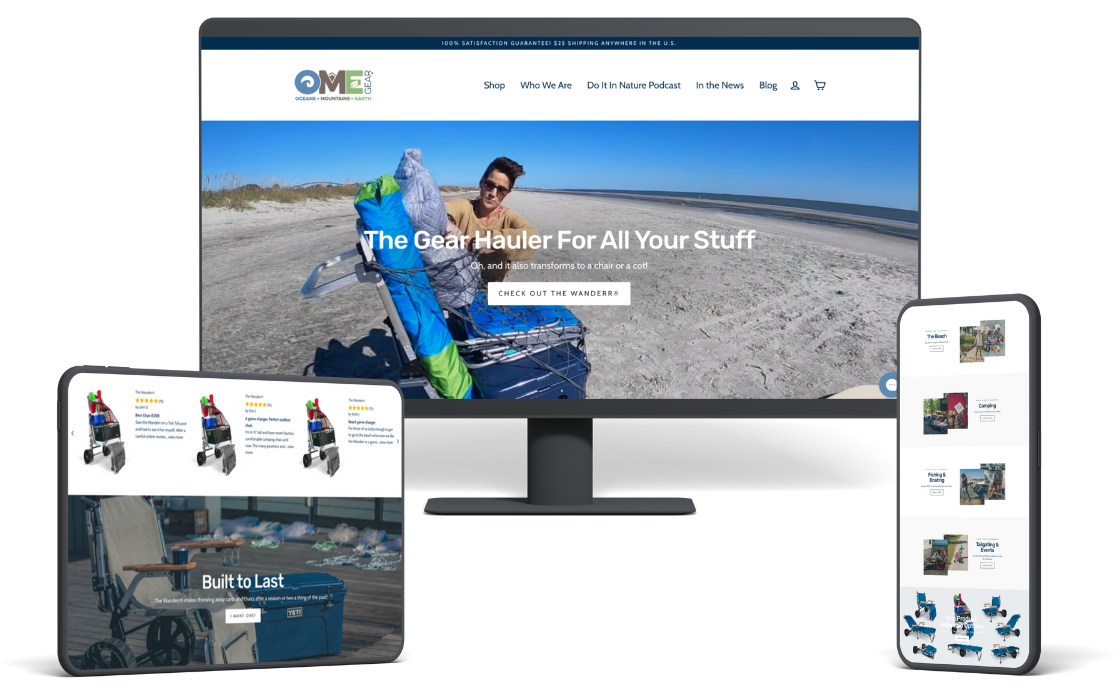The image showcases the website interface of a specialized travel and extreme sports retailer named "OMEGA." Displayed on a computer monitor, tablet, and phone, the website emphasizes customer satisfaction and convenient shipping options, prominently stating "100% Satisfaction Guaranteed" and "$25 Shipping Anywhere in the US," indicating it's a US-based site.

The home page on the computer monitor includes navigation options such as "Shop," "Who We Are," "Do It in Nature Podcast," "In the News," "Blog," personal account access, and a shopping cart. 

Featured on the page is an image of a man equipped for an adventure, standing on what appears to be a desert or beach, under a vibrant blue sky. He is wearing glasses and has a prominent quiff hairstyle. The spotlight product shown is a versatile "Gear Hauler," which intriguingly transforms into a chair or cot. Above the image, the caption "Check out the wonder" is creatively spelled with two R's, adding a unique touch to the promotional content.